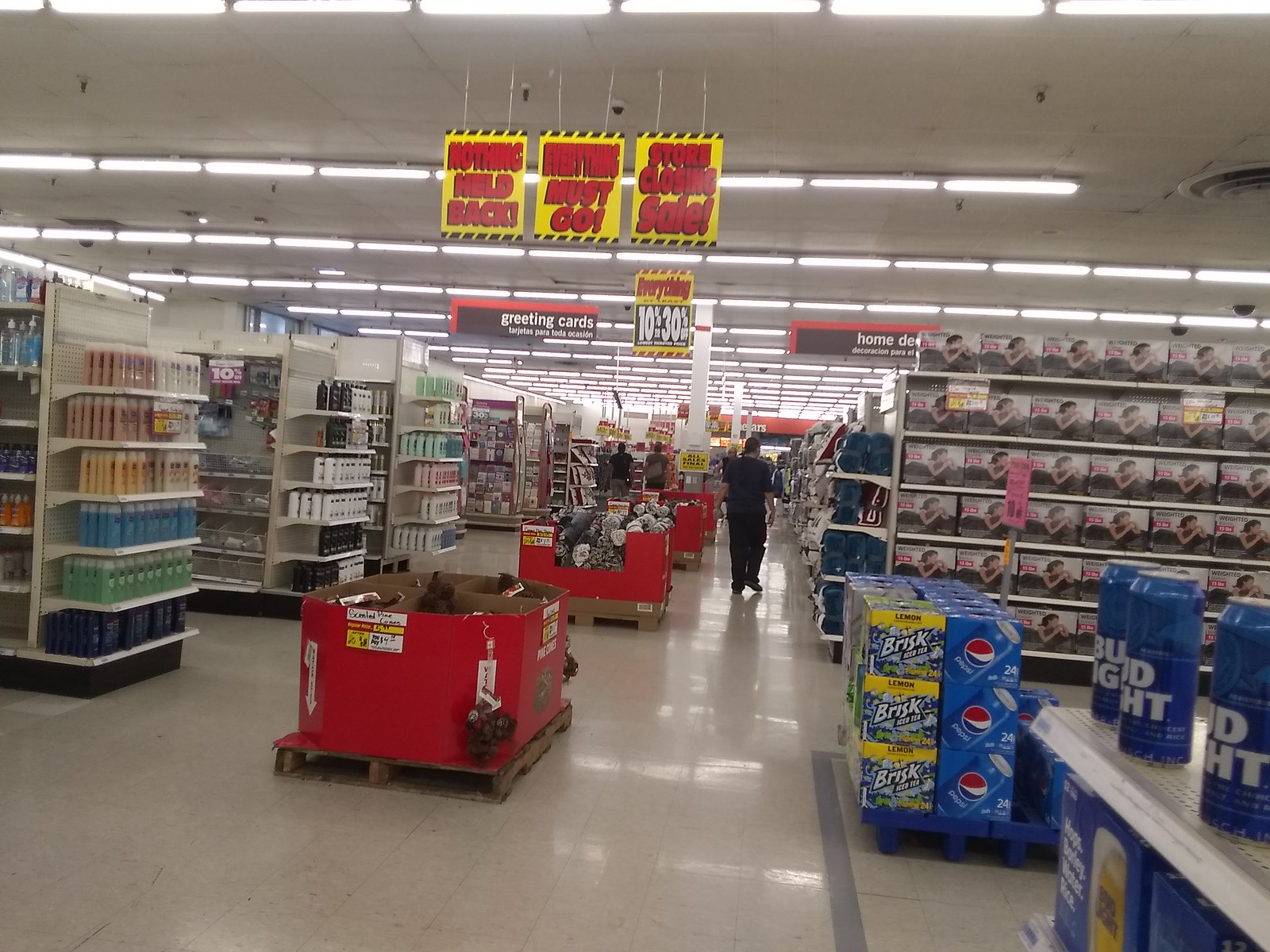This vivid color photograph captures the interior of a bustling shopping store or mall. The ceiling is adorned with large, bright fluorescent lights set against a grey background. Central to the image are vibrant yellow signs with red text, most likely advertising special offers or promotions, although the exact wording is unclear.

Prominent shelves brimming with products extend across the scene. On the left, rows of bottles suggest they may be personal care items such as shampoos or conditioners. Dominating the middle area are red storage bins filled with various goods. The nearest bin appears nearly empty, while the one behind it contains indistinct grey objects.

To the right, more shelves hold boxed items whose details remain obscured. In the lower-left corner, a shelf is stocked with blue cans labeled with white letters, partially spelling out "0" and "HT." Above these, additional shelves display brightly colored cartons, some labeled with the word “bright” in hues of blue and yellow. These cartons bear a striking resemblance to Pepsi products, distinguished by their blue coloring and red-and-white circular logos.